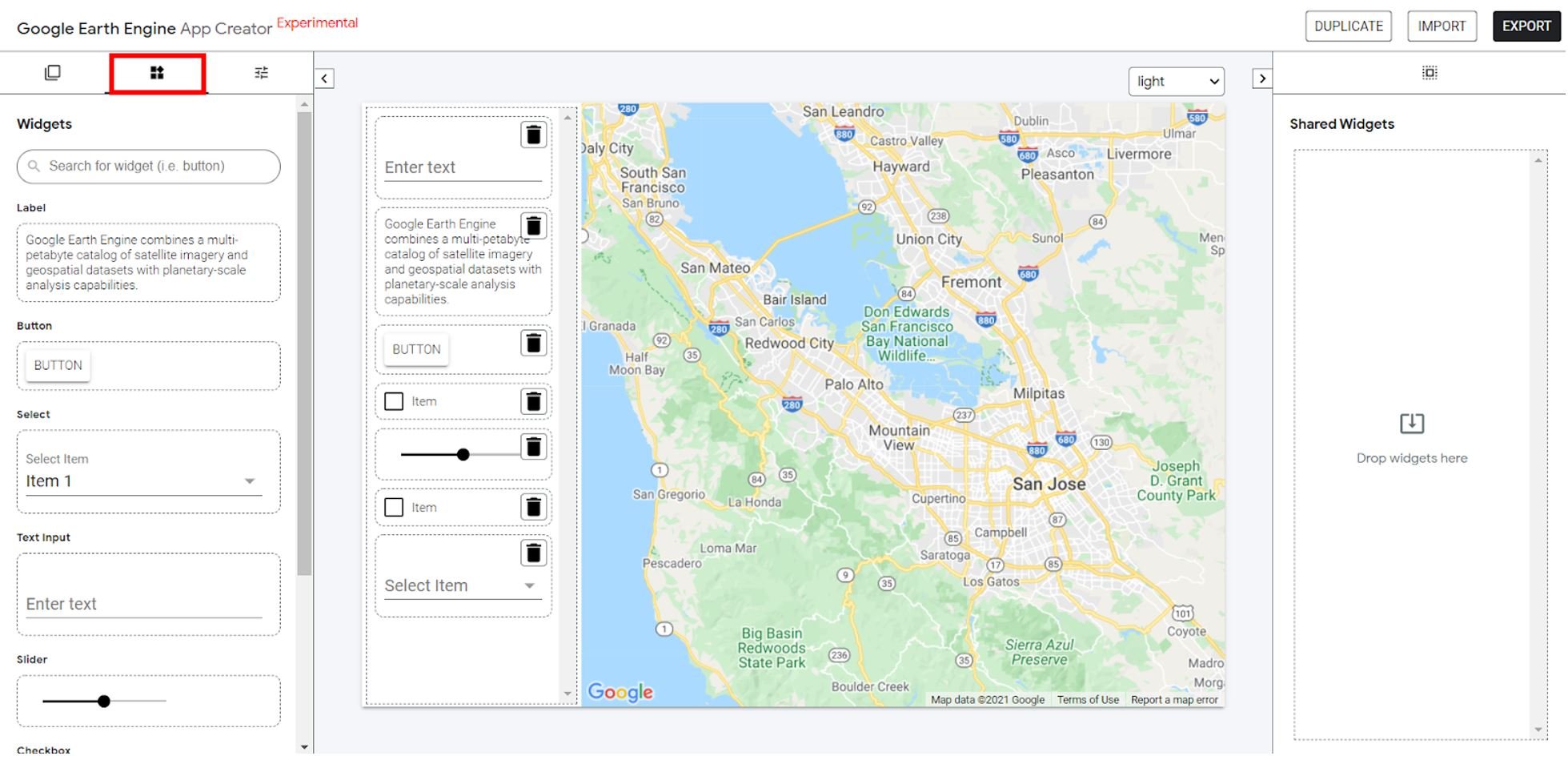The image is a screenshot taken from the Google Earth Engine app creator, displayed on a white background. At the top left corner, the name of the program is visible, alongside a red label indicating that it is "experimental." Below the program name, there is a black outlined box with three category options, each represented by various icons. The middle option is selected, noted by a red outline around it. 

Further down within this section, we see subcategories labeled "widgets," and a search option that includes the hint "IE button" in parentheses. Additional subcategories are listed below, including label, button, select, text input, slider, and checkbox, though not all are fully visible due to cropping.

Moving to the right-hand side, there is a colorful map of a region in California. Adjacent to the map, on its left, there is a text entry field. The interface illustrates Google Earth Engine's capabilities of combining a vast multi-petabyte catalog of satellite imagery and geospatial data sets with planetary-scale analysis tools. Below the map, there are options such as a button, an item, a slider scale, another item, and a dropdown select item.

On the far right side of the image, another section is delineated by a white background. This area, labeled "shared widgets," allows users to drop widgets into the area. Above this section are three buttons: "duplicate," "import," and "export." The "export" button is black with white text, while the "duplicate" and "import" buttons are white with black outlines and black text.